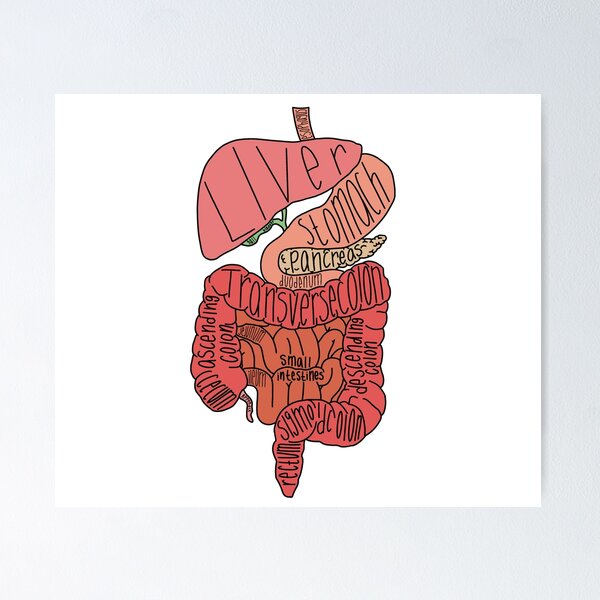The image is a detailed illustration on a white square canvas, featuring labeled internal organs with an artistic touch. Set against a light gray background with a slight drop shadow to the right, the organs are drawn in black ink and filled with various colors, including light pink, beige, salmon, brown, and green. The liver is illustrated in green, connected to the stomach, and prominently labeled "liver" with text that fills its interior. Below the stomach, also labeled, lies the pancreas. The large intestine, depicted in red, wraps from the left side upward, crosses under the stomach and pancreas, makes a 90-degree turn downwards, and transitions into the rectum. The illustration also labels the ascending colon, transverse colon, descending colon, and sigmoid colon, with small intestines intricately snaking within the large intestine. Overall, the drawing meticulously portrays the liver, stomach, pancreas, colon segments, and intestines, emphasizing their connections and anatomical positions.